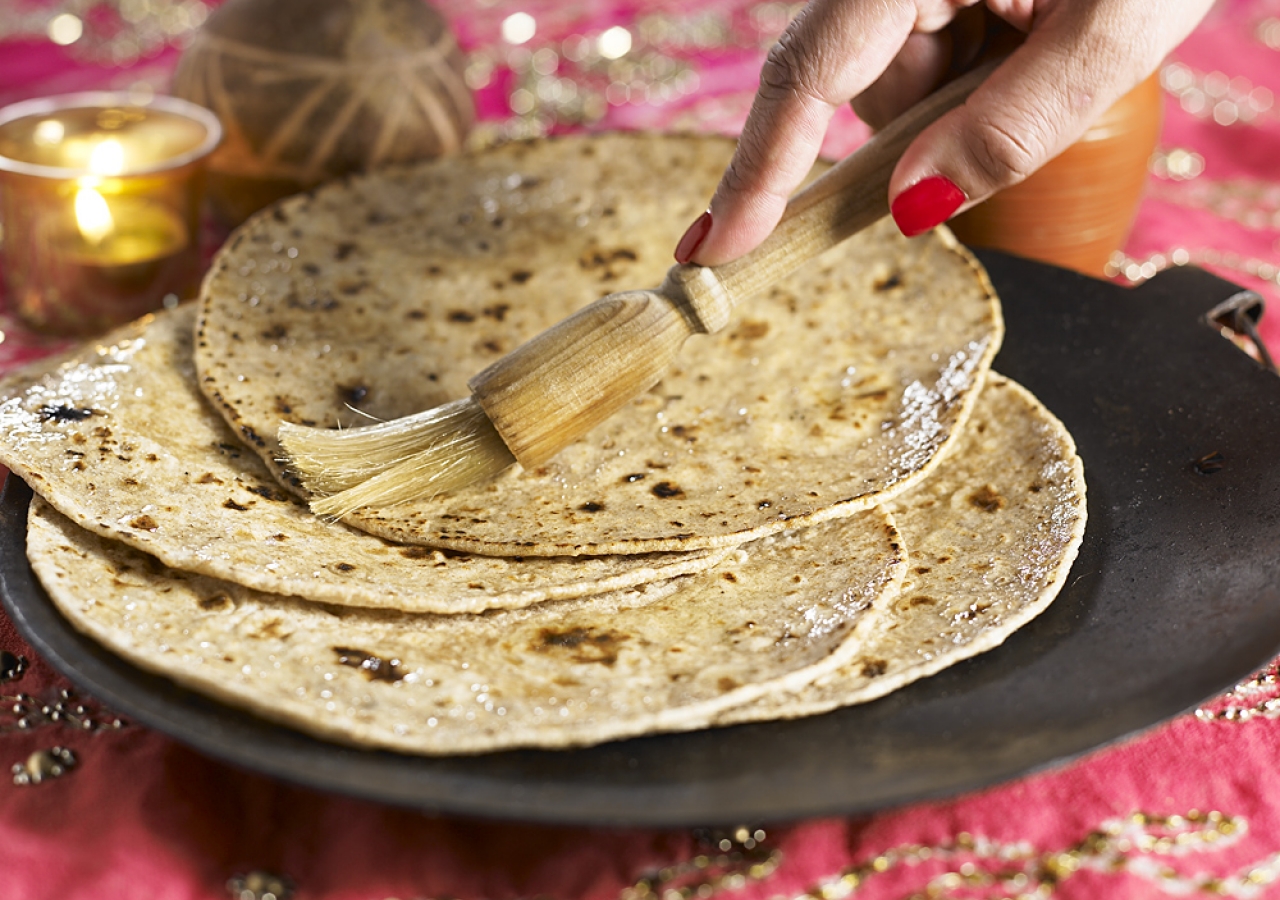The image depicts a close-up of a woman's hand with red nail polish, using a wooden cooking brush to apply a clear, shiny oil onto a stack of four soft tortilla shells or flatbreads. The flatbreads are slightly charred and stacked unevenly on a curvaceous brown or black plate that might have a ring handle on one side. This setup is placed on a table adorned with a pinkish-red tablecloth interwoven with intricate gold accents and patterns. In the background, there is a lit tea light candle in a votive holder, a goldish cup, and a reddish-orange vase, adding to the overall warm and cozy ambiance of the scene. The table setting suggests a meal preparation or serving activity in progress.